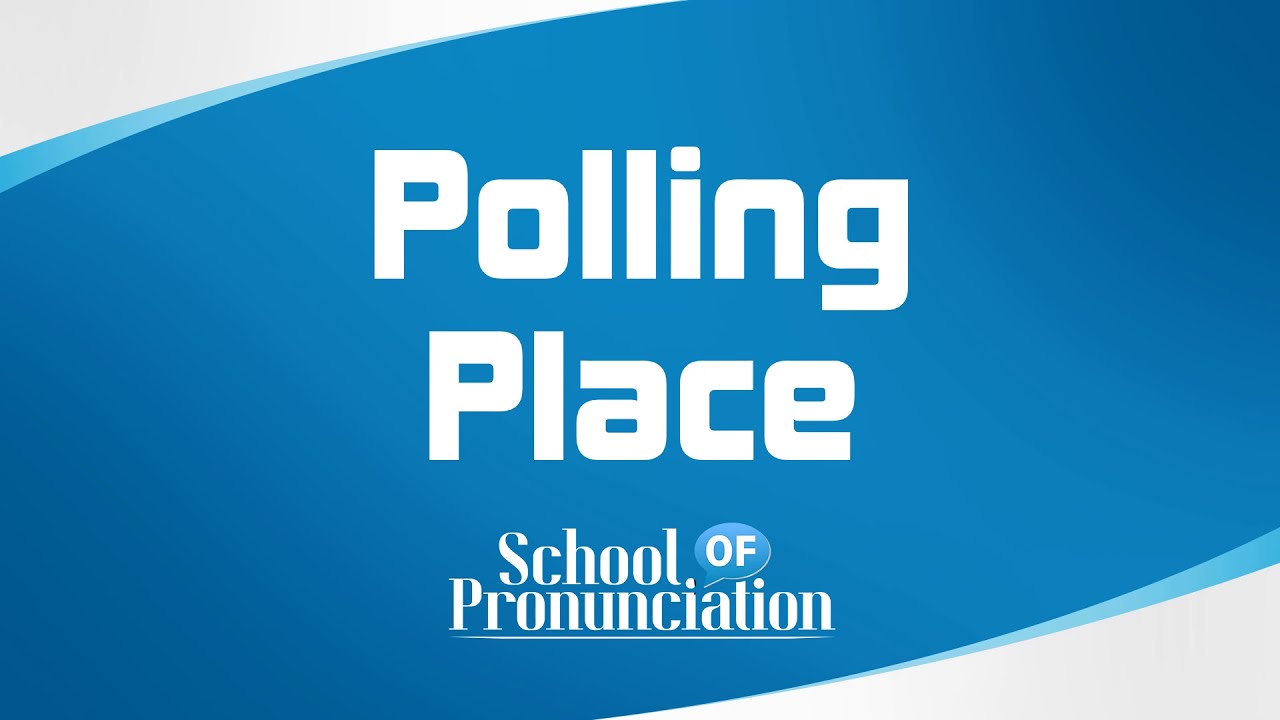The image is a horizontal rectangular graphic with a dark blue background that stretches diagonally from the upper right corner to the lower left corner, leaving off-white edges in the bottom right and upper left corners. The dark blue area has a pale, light blue outline that adds a three-dimensional effect. A slanted light blue arc inside the dark blue space becomes more pronounced as it extends toward the edges. In the center, large bold white letters read "Polling Place." Directly beneath, smaller white letters say "School" followed by the word "of" enclosed in a light blue speech bubble. The text "Pronunciation" follows, underlined with a white line. The image appears to serve as an advertisement or a slide, possibly for a PowerPoint presentation.